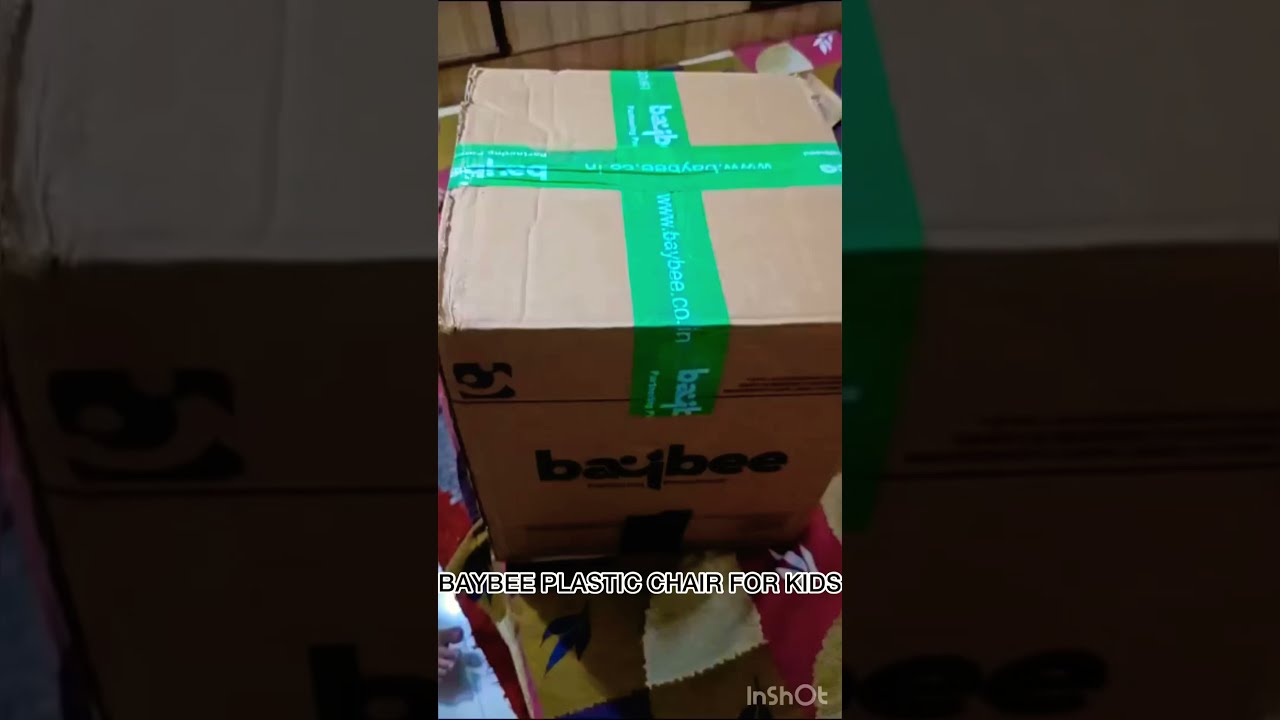This image features a top-down view of a cardboard box, which appears in the middle third of the image. The box is light to medium brown, roughly cubic in shape, and sealed with green packing tape that forms a cross on the top. The tape has white text that reads "www.baybee.com," with the website name "B-A-Y-B-E-E" also visible on the side of the box. The side of the box also features the word "baby" in black print.

Superimposed on the left and right thirds of the image are zoomed-in, dimmed, and blurrier sections of the same original picture, providing a mirrored and border-like effect. Below the box, towards the bottom right corner of the main image, the app name "InShot" is displayed in white text, while the words "Baby Plastic Chair for Kids" are written below the box in black font with a white outline.

The box sits atop a multicolored pile of cloth or clothing, featuring patches of yellow, red, white, blue, and brown with no discernible pattern. The background reveals a brown wall, and barely noticeable in the lower left corner are someone's bare toes.